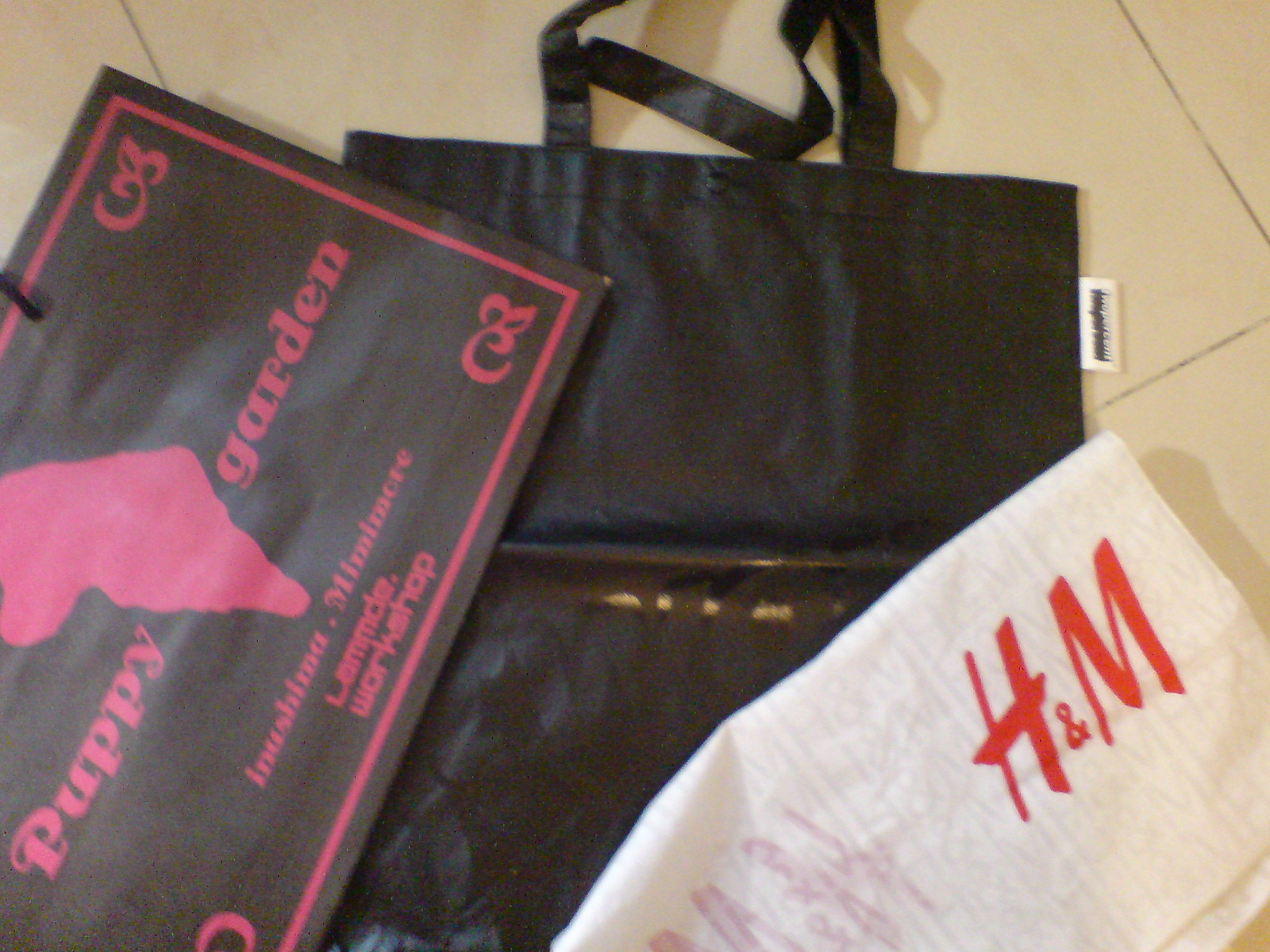The image depicts three distinct items arranged on a tan-colored tiled floor, characterized by visible black mortar lines. At the center is a black fabric bag with two handles, partially obscured by other objects. On top of this bag lies a folded white bag, prominently displaying the bright red letters "H&M" in the upper right corner. Adjacent to it, also placed on the black bag, is a piece of paper that reads "Puppy Garden" amid some indistinct text and features an image of Africa. The composition highlights the three items—the white H&M bag, the black fabric bag, and the "Puppy Garden" paper—set against the neutral tiled flooring.